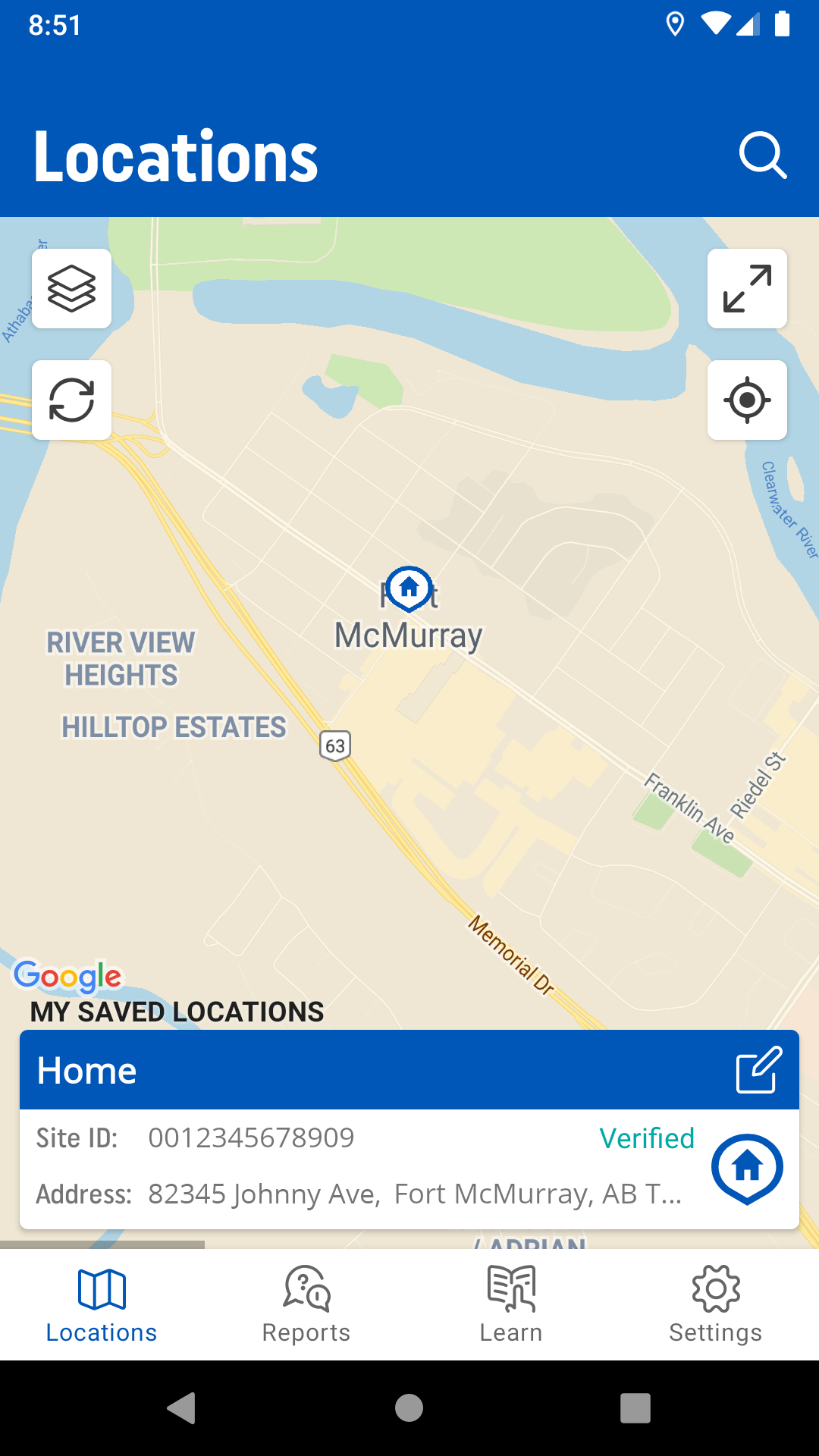The image is a screenshot of a smartphone displaying the Google Maps application. The image appears to be about two to two and a half times taller than it is wide. At the very top left of the screen, the time reads 8:51 in white text. On the top right corner, there are icons indicating signal strength and battery level, confirming it is a mobile device.

A blue banner occupies approximately 15 to 20 percent of the upper portion of the screen. Within this banner, the word "Locations" is prominently displayed in bold white letters on the left side. On the lower right edge of the banner, there is a magnifying glass icon, suggesting a search function.

The main section of the image is a view of Google Maps. It displays various standard elements such as zoom and refresh icons at the top, and the "Google" label at the bottom, indicating authenticity. A specific location, marked with a pin and labeled "McMurray," is highlighted. Beneath the map is another blue banner labeled "Home," indicating a saved location. To the right of this banner, there is an edit option. Below, additional details such as a site ID and an address are presented, with a "Verify" option on the right.

At the very bottom of the screen, icons for navigation through the app are visible, including "Locations," "Reports," "Learn," and "Settings."